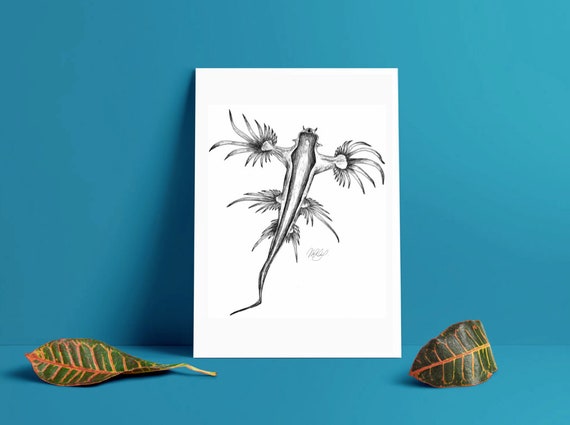The photo showcases a richly detailed, black and white pencil sketch of an enigmatic, fish-like creature set against a vivid turquoise backdrop. The creature appears to have a slender body that widens at shoulder level, reminiscent of a dragonfly, and tapers down into a long, curving tail. At its top, the creature possesses tiny antennae or whiskers, giving it an alien and oceanic vibe. The body features multiple extensions including two sets of fin-like, leg-like appendages that branch out into long, wavy, seaweed-like forms or leaf-like feathers, enhancing its exotic appearance. The sketch is rendered on a white piece of paper standing upright against the turquoise wall, with the same turquoise color extending to the floor. Adding to the tropical aesthetic, the bottom corners of the paper are framed by two large, curling green leaves, distinguished by their striking orange and red veins. This intricate and otherworldly artwork, reminiscent of a dangerous aquatic creature, anchors the composition of the fascinating and surreal image.